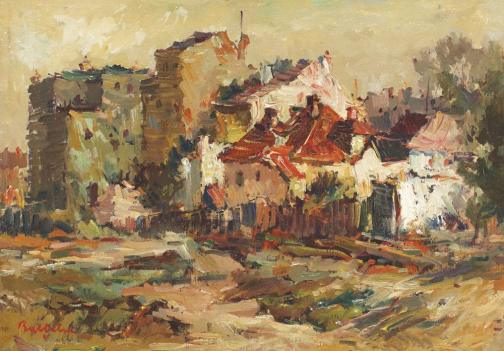This image showcases an impressionistic painting of a small village with a cluster of buildings of various sizes and colors, each rendered in a loose and abstract style. The foreground features a landscape characterized by green grass, swamp bushes, and brown brushstrokes representing dirt. Intricately painted, a dark and light brown wooden fence stretches across the middle, framing the village scene. Dominating the village, there is a prominent greenish three-story building. To its right stands an orangish building, followed by a pinkish one. Below these structures, two smaller buildings with orange roofs and a yellow-orange facade are visible. The rightmost structure is a white house with a light tan roof. The village comprises one-level houses with pitched roofs and larger, rectangular buildings that resemble apartments or offices with flatter roofs. The sky looms gently behind the entire scene, highlighting the serene, pastoral setting.